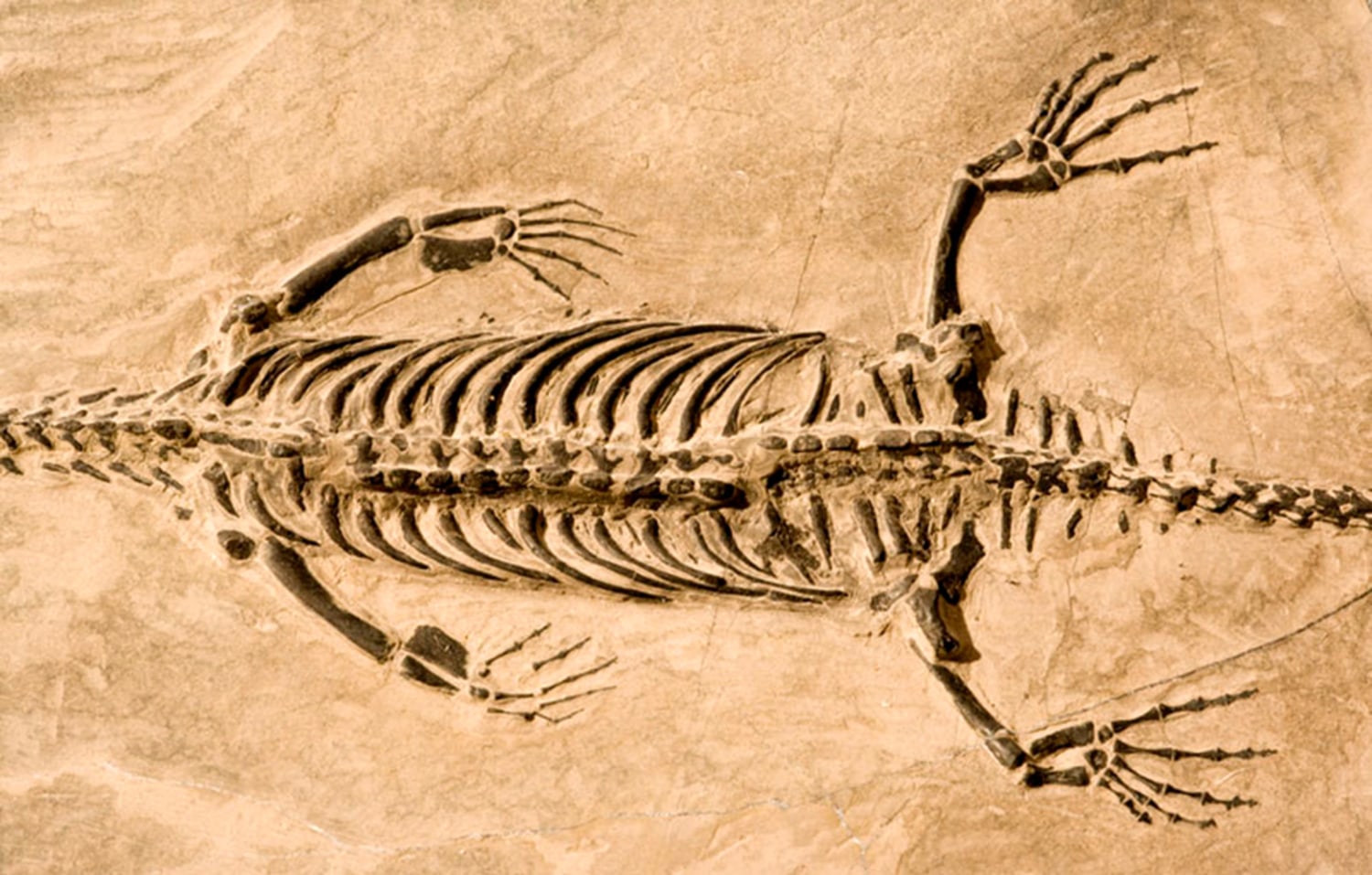This photograph captures the fossilized remains of a reptilian-like animal, potentially a dinosaur, embedded in a sandy, tan, and beige rock. Positioned centrally in the image, the fossil displays an extraordinary level of detail with individual vertebrae, ribs, and bones meticulously preserved. The skeleton, dark in color against the lighter rock, appears to have been in a prone position at the time of fossilization. The animal’s four limbs, each revealing five fingers or toes, are clearly visible, although parts of the tail and head are missing or cut off, suggesting some damage, particularly near the tail section and back limbs. The well-lit setting suggests the photo was taken on a sunny day, enhancing the natural earthy tones and the remarkable condition of the fossil despite some visible damage to the neck and shoulder regions.